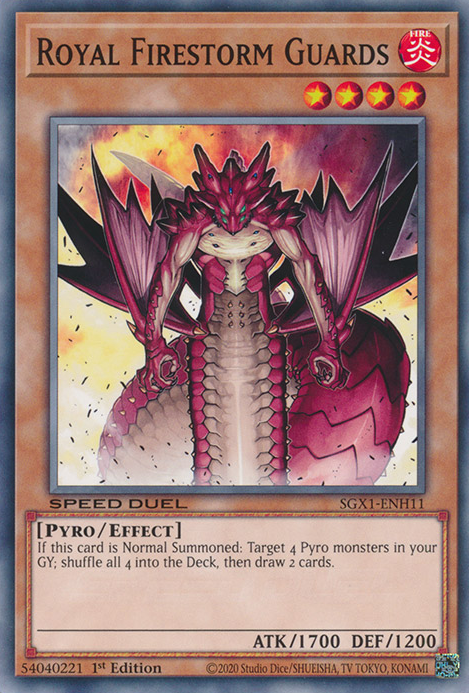The image depicts a trading card, which appears to be part of a gaming set similar to "Magic: The Gathering." The card, titled “Royal Firestorm Guards,” features a central illustration of a large, muscular, reddish-pink creature with a snake-like body, wings, two arms, and a head adorned with multiple horns. This creature is set against a backdrop of intense yellow and orange flames. Surrounding the title “Royal Firestorm Guards” at the top, there are four red circles each containing a yellow star. Below the image, the card details its abilities and features. It reads “Speed Duel SGX1 ENH 11” with a “Pyro / Effect.” The card’s specific ability states: “If this card is normal summoned, target four Pyro monsters in your GY, shuffle all four into the deck, then draw two cards.” At the bottom, the card provides stats: ATK 1700 and DEF 1200. The overall card design includes a brownish-marble background contributing to its thematic aesthetic.